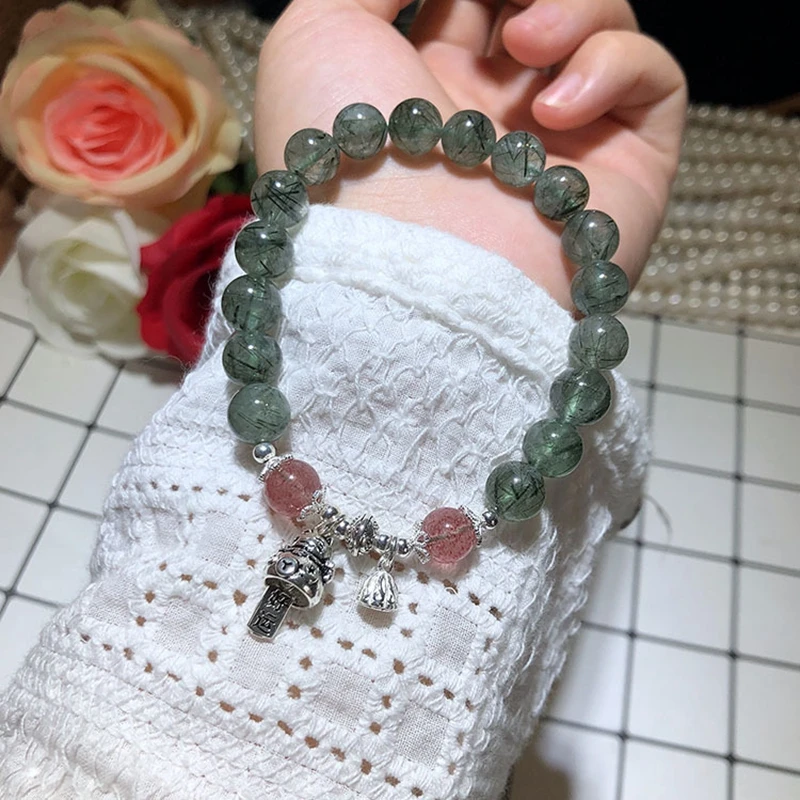The image features a detailed close-up of a young woman's arm and hand, covered by a white knitted sleeve extending just beneath the elbow to the wrist. The hand is palm-up, displaying a rosary that rests gently on the wrist. The rosary is composed predominantly of greenish-gray glass beads, with the two beads closest to the end standing out in pink glass. It is attached to a silver Celtic-style crucifix, accompanied by several other silver charms, including a small bell and a decorative medallion. The aesthetic arrangement includes three roses positioned to the left of the arm: a vibrant red rose, a pure white rose, and a pinkish-orange rose, enhancing the visual contrast between the green glass beads and the white blouse. Small pearls are also scattered nearby, completing the elegant scene.